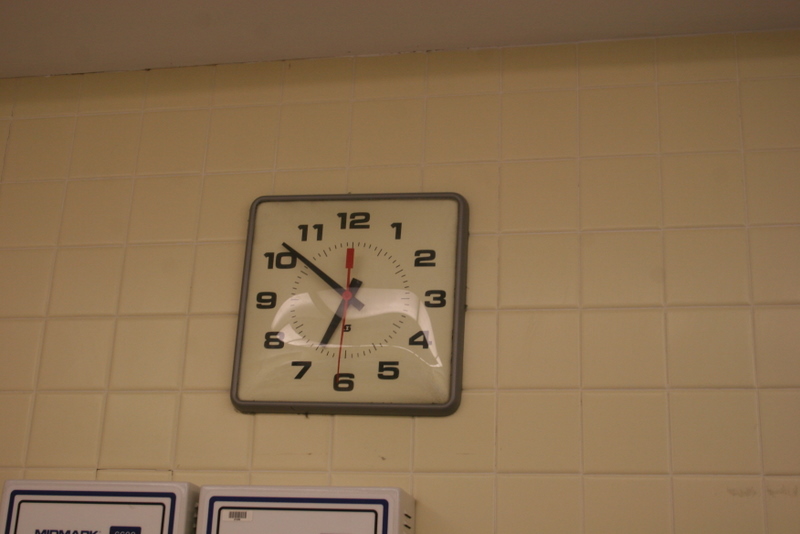A detailed image caption could read:

"A square wall clock, with an off-white face, black numbers, and black hour and minute hands, hangs prominently on an off-white, square-tiled wall. The second hand is red and points slightly beyond the 6, indicating 31 seconds past. The time displayed on the clock is 6:51. In the lower left-hand corner of the image, the tops of some white and black boxes are visible, also mounted on the wall. A partial view of a white ceiling is seen in the top left corner, with a shadow extending across the ceiling and cascading halfway down the first row of tiles. Additionally, there is a light reflection on the clock face, adding depth to the scene."